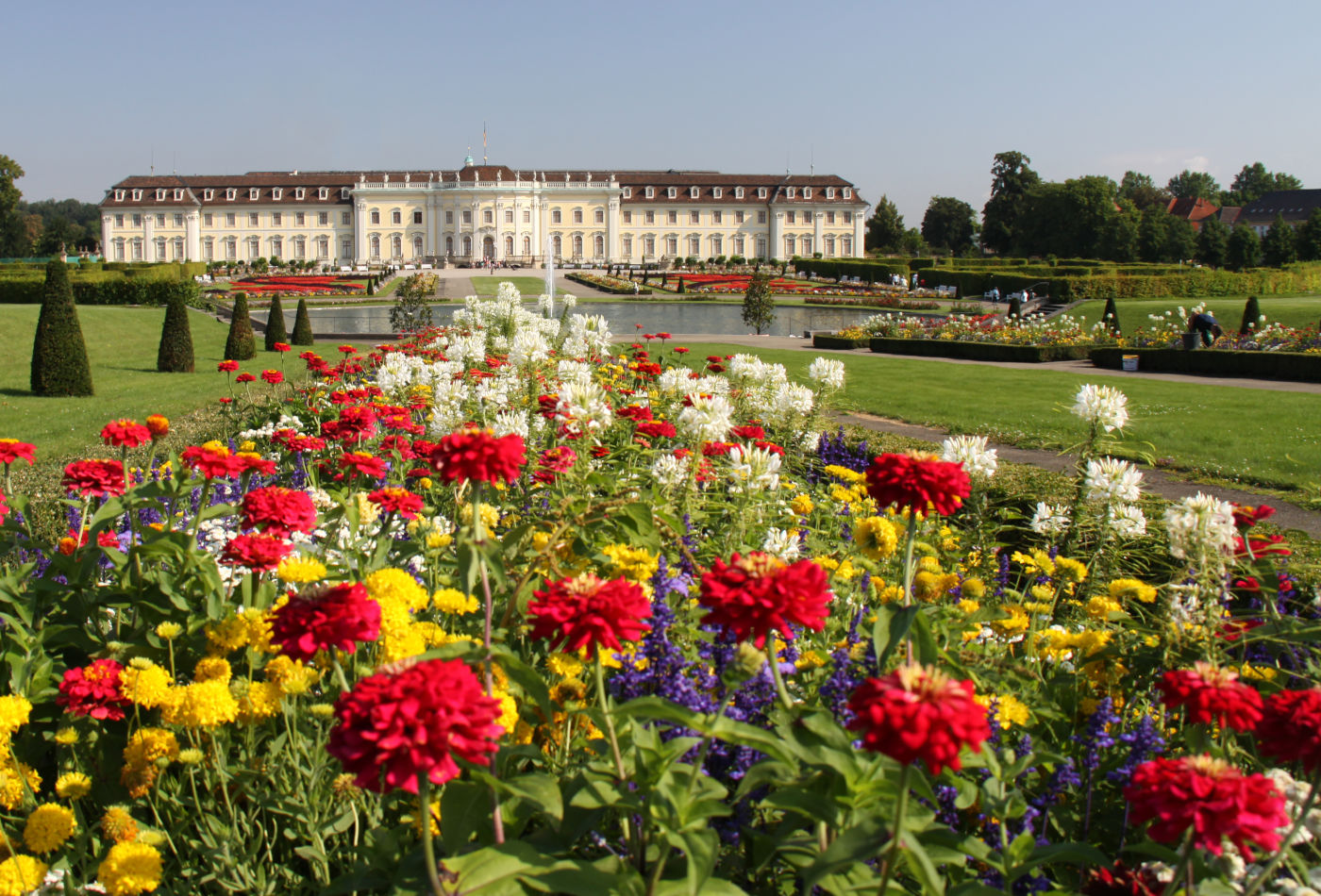The photograph depicts a stunningly ornate and formal mansion bathed in daylight, set amid an expanse of precisely manicured gardens. In the foreground, a vibrant array of flowers—red, yellow, white, and purple—adorn lush green stems and leaves, providing a rich tapestry of color. Further back, immaculate lawns and landscaped gardens stretch out, peppered with shrubs and additional flower beds. A round decorative pool, approximately 100 feet in diameter, graced with a small central fountain, adds to the elegance of the scene. The mansion itself, towering two to three stories high, features white and beige creme walls, punctuated by a brown Mansard-style roof. Its architectural elements, reminiscent of classic European or American design with pillars and rounded facades, exude grandeur and officialdom. The setting suggests it could be either a prestigious private residence or a significant government building. Trees encircle the mansion, contrasting beautifully against the clear blue sky, which is free of clouds, casting a serene and picturesque backdrop to the floral foreground and verdant lawns.